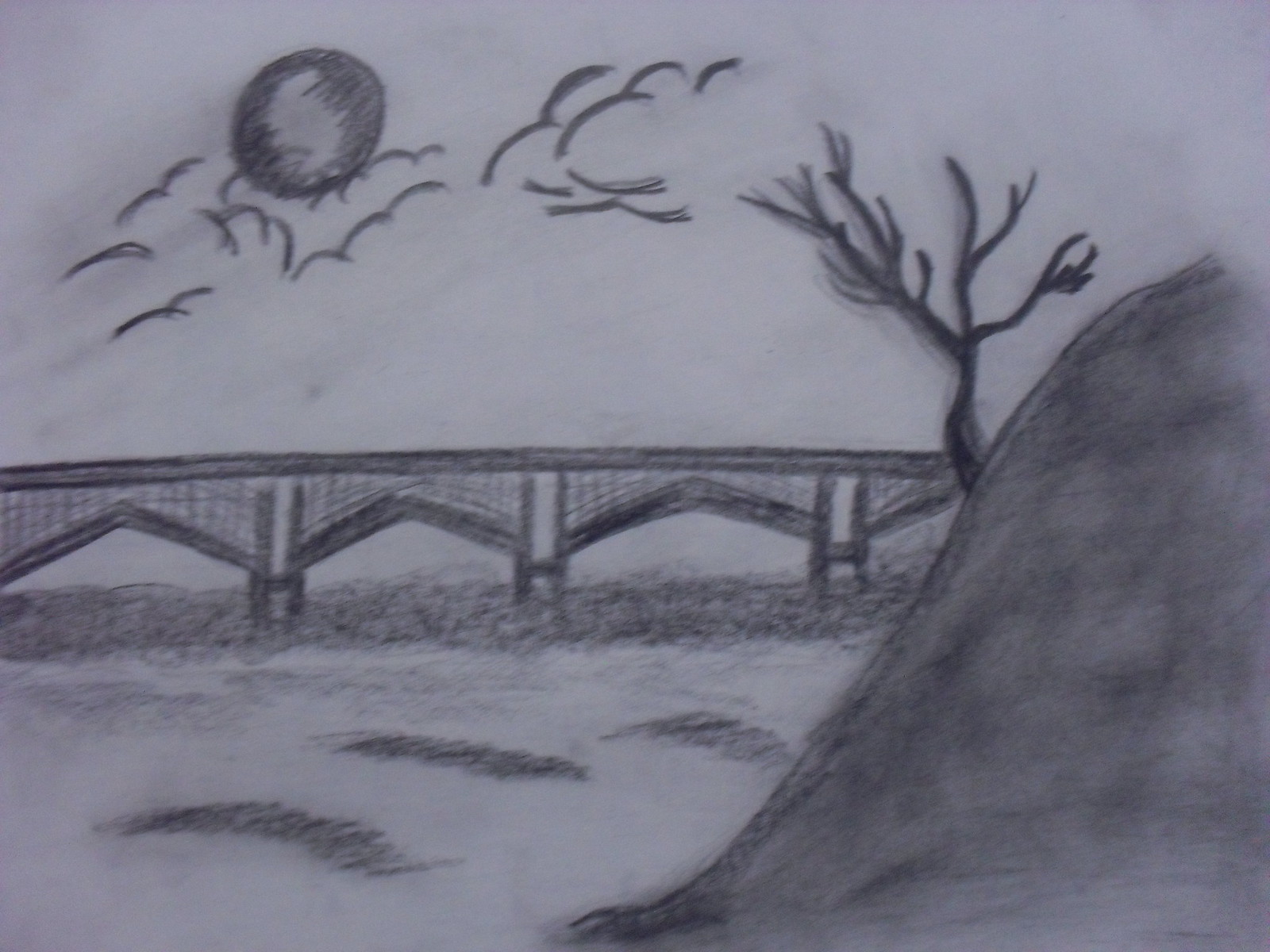This black and white drawing, which appears to be a proficient work by a possibly young artist, depicts a serene scene dominated by a large hillside on the right side. Atop the hill, a leafless tree stretches its branches outward. Emerging from the base of the tree, a detailed bridge spans across a body of water, resembling a bay or river mouth, toward the left side of the image. The bridge is supported by a series of metal frames, shaped like upside-down Vs, with each support structure intricately lined with numerous wires, while the roadbed is marked by a double penciled line filled in with gray.

The sky above is filled with elements that add a sense of depth and intrigue: clouds or bird-like forms are sparsely drawn, and a prominent shaded circle, likely the moon, floats near the top left. Bats can be seen scattered around this celestial object. On the hillside, the terrain descends diagonally to the left and off the bottom of the page, contributing to a balanced composition. Below the bridge, the water reflects subtle wave patterns, enhancing the tranquil atmosphere of this meticulously crafted scene.